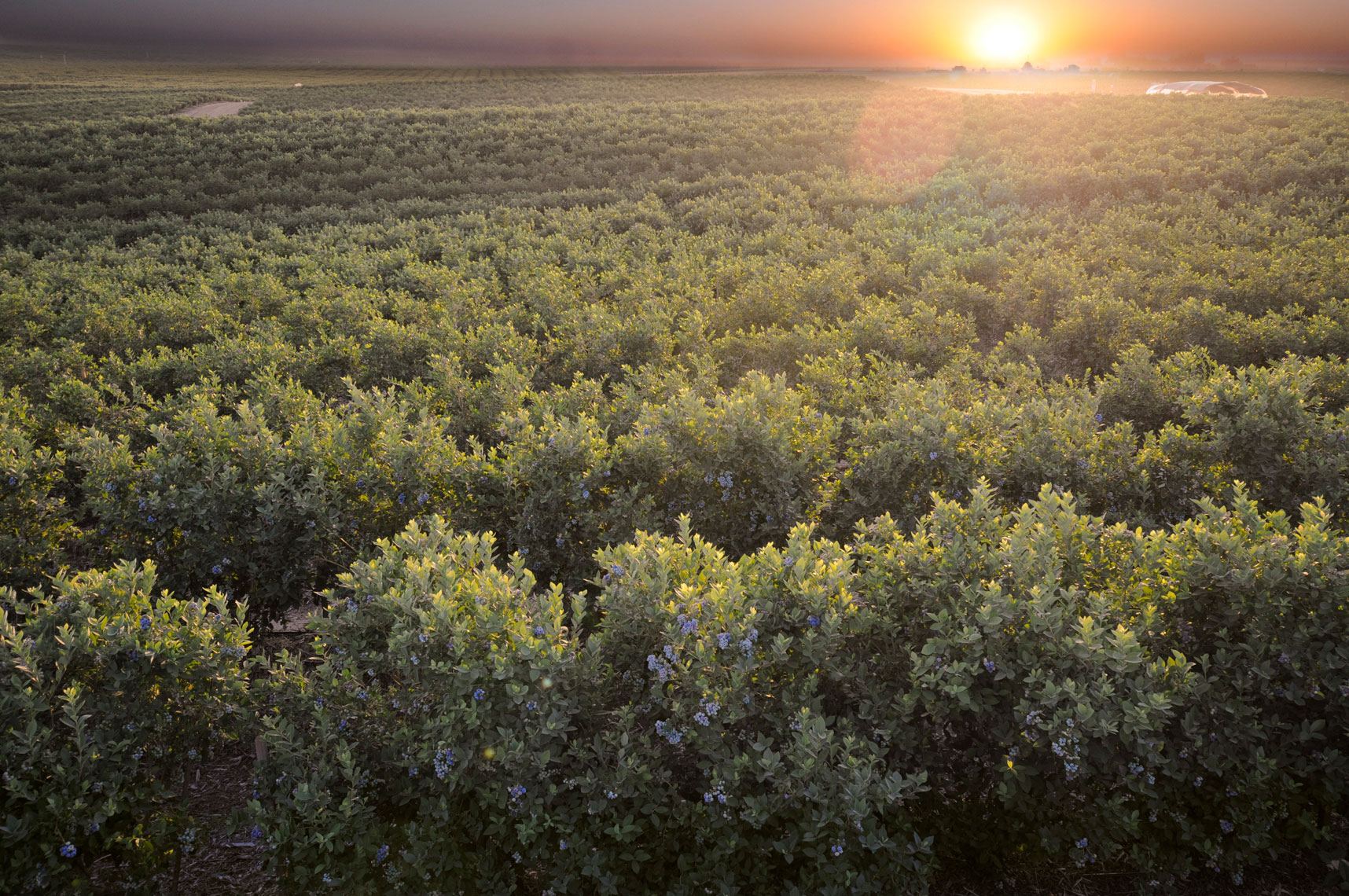This horizontal, rectangular photograph artfully captures what appears to be a sunrise or sunset over a neatly cultivated field of rosemary bushes, characterized by their blue flowers and short, skinny leaves arranged in organized rows. The field features a slight diagonal tilt, with shadows accentuating the spaces between plants. The landscape is mostly flat with minor undulations, creating subtle shadowy dips. In the middle right, a glowing, spherical sun emits a soft orange light, contrasting with the darker grey clouds that dominate the upper left sky. A circular spot near the bottom left of the sun hints at a lens flare. Faint structures add depth to the scene: a possible concrete foundation or building in the upper left, and a row of sunlit buildings and trees beneath the sun in the upper right. Overall, the image combines green foliage, yellow sunrays, and orange hues to create a harmonious, almost surreal portrayal, leaving one to wonder if it’s a painting or an exceptionally captured photograph.